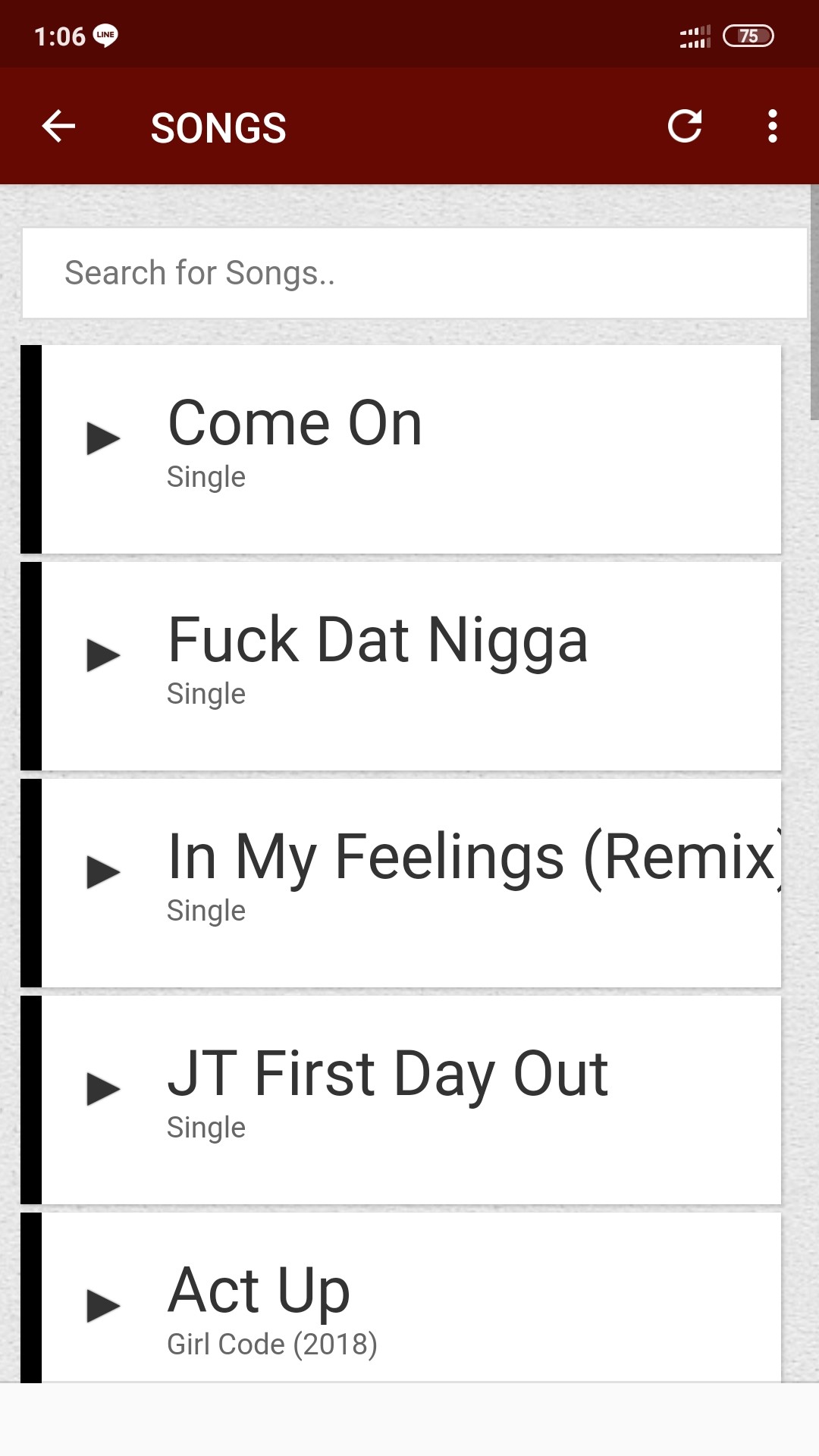A screenshot taken from a phone displaying a music app interface. The top section features a blank background with a white text on the left showing "106" and next to it, a speech bubble icon with the word "wine" inside. Below this, there are two cell phone signal indicators and a circle with the number "75" inside. To the left of this circle is a back arrow icon labeled "songs," and on the right, there are refresh and menu (three dots) icons.

The background below this section is entirely gray. Centrally placed on this gray background is a white search box with gray text that reads "search for songs." Below the search box, there are five rectangular sections, each featuring a black triangle pointing to the right, resembling a play button. The boxes are predominantly white with a small black streak on the left side.

The listed songs in these sections are:
1. "Come On" labeled as a single.
2. "Fuck Dat Nigga" labeled as a single.
3. "In My Feelings Remix" labeled as a single.
4. "JT First Day Out" labeled as a single.
5. "Act Up" labeled under the "Girl Code 2018" album designation. 

The overall interface is minimalist and functional, focusing on song selection. However, some of the song titles contain explicit language.